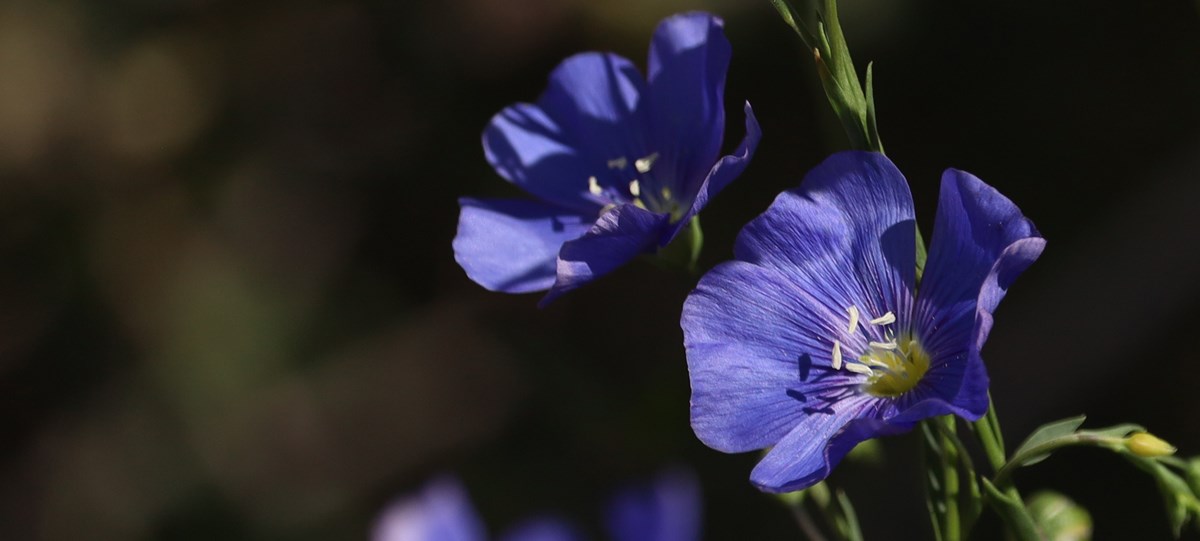This image, a color photograph in landscape orientation, captures two prominent morning glory flowers set against a very dark background. The image is zoomed in closely, giving a detailed view of the blossoms. The flowers, with their fluted petals, are a purple-indigo color that varies in shade from light to dark across the petal surfaces. The top flower, placed towards the center at the top, is partly in shadow, while the lower flower, closer to the viewer, faces the left center. Each blossom features a cluster of wispy green and white stamens at its center, along with a few yellow stamens.

The arrangement of the flowers reveals a delicate ruffle at the edges of the petals, adding to their intricate appearance. The flowers are attached to a dark green vine that diagonally traverses the image from the bottom right toward the top left. This vine is adorned with a few bumpy, not smooth, leaves curled underneath the bottom right. Additionally, there are more out-of-focus purple flowers along the bottom, hinting at a fuller scene beyond the immediate focal point.

The overall setting is characterized by its out-of-focus dark background, creating a stark contrast that highlights the vibrant flowers. No text or people are present, ensuring the viewer’s focus remains on the botanical beauty depicted with photographic realism.